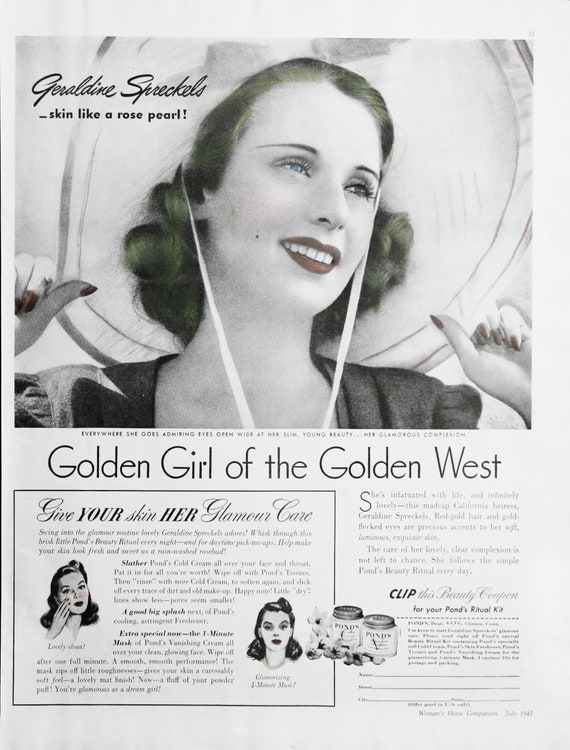This black and white 1920s or 1930s newspaper clipping is an old skincare advertisement featuring Geraldine Spreckels, hailed as the "Golden Girl of the Golden West." Dominating the ad is a striking image of Geraldine, a woman with a pale complexion, vivid red lipstick, and matching red nails. Her stylish appearance, reminiscent of Marilyn Monroe, is accentuated by a large sun hat and slightly tinged greenish hair, which subtly contrasts the grayscale backdrop. Geraldine gazes upwards and to the side with a smile, exuding an air of glamour. The ad headline proudly proclaims, "Geraldine Spreckels, Skin Like a Rose Pearl," and urges readers to "Give your skin her glamour care." Below is a detailed skincare regimen recommendation involving a Pond's product, complete with a small inset image depicting a two-step application process: Geraldine first applying the cream and then showing her face covered with it. To the bottom right, there is a call to action to "clip this beauty coupon for your Pond's Ritual Kit," accompanied by a visual of the actual Pond's product, enhancing the viewer's understanding of the skincare solution promoted.